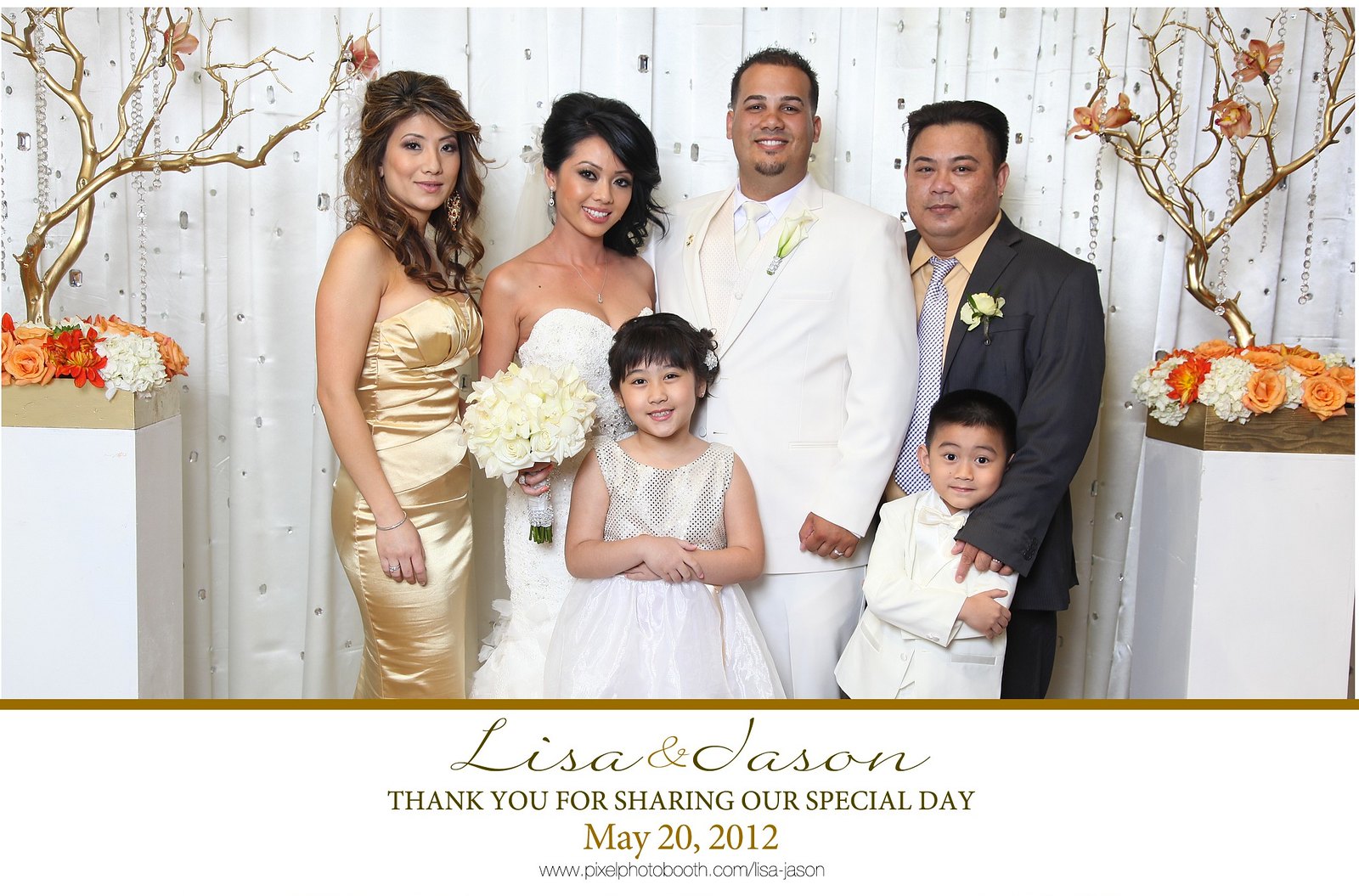In this wedding photograph, six people are elegantly posed in front of a white curtain adorned with crystals. White planters on either side feature orange and white flowers, with golden tree branches sprouting from them. On the far left stands a beautiful woman with long brown hair, dressed in a strapless gold gown. Next to her is the bride, radiant in a strapless white gown, holding a bouquet of white flowers, with her dark hair swept over her right shoulder. A young girl in a white sleeveless dress, with her dark hair pulled back, stands in front of the bride. The groom, positioned next to the bride, looks dapper in an all-white tuxedo with a yellow rose in his lapel. He has short spiked black hair and a goatee. To the right of the groom stands a man in his fifties, wearing a gray suit, an orange shirt, and a blue and white dotted tie, also with a flower in his buttonhole. In front of him is a young boy in a white tuxedo with dark hair. An inscription below the photo reads, "Lisa and Jason, thank you for sharing our special day. May 20, 2012."